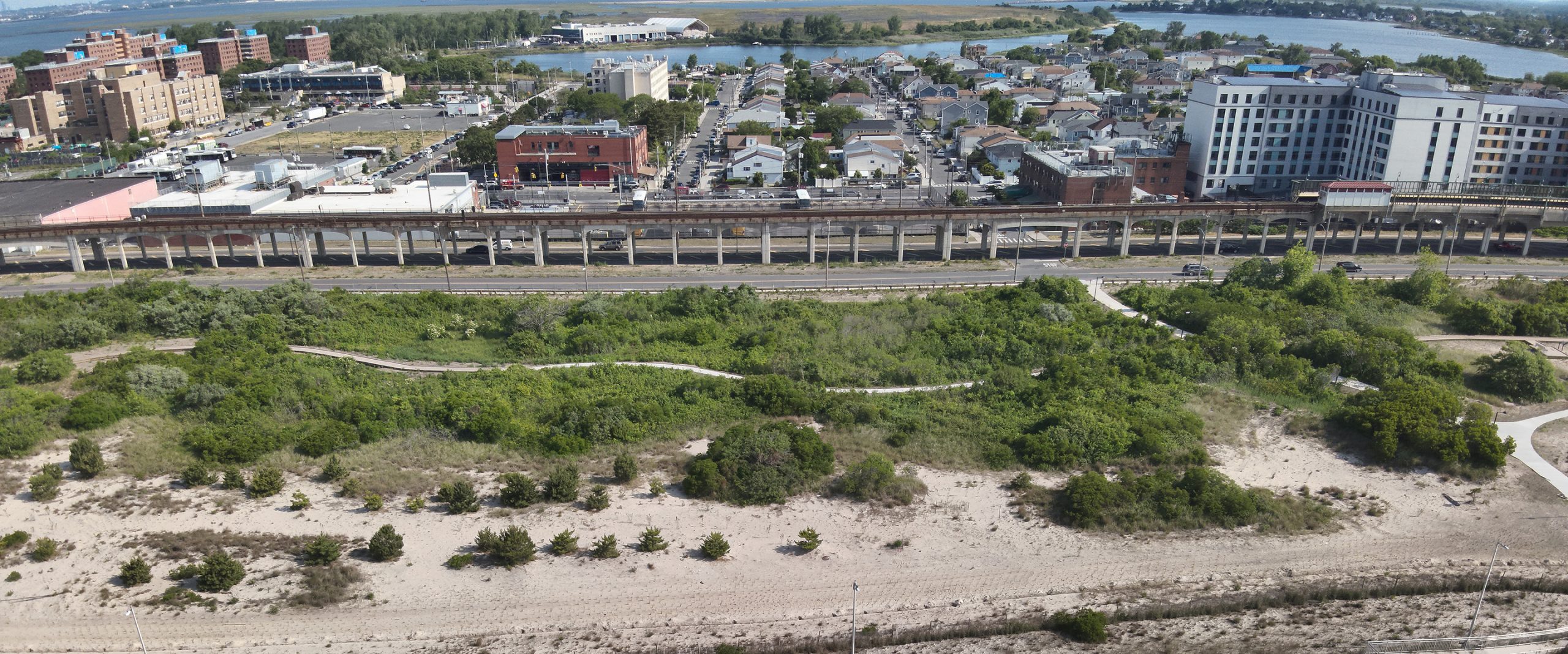This aerial image captures a quaint coastal town, likely situated in either Florida or the Carolinas, during the late afternoon. The foreground features a sandy, natural beach that appears unmanicured and overgrown with lush greenery, forming a pathway to the water's edge, which is not visible in the image. Just beyond the beach lies a sparse road with one or two cars, paralleled by a raised railway track.

The midground reveals a series of diverse buildings, including white and red brick houses with red shingle roofs, interspersed with modern residential and commercial structures. Notable among these is a white-painted hotel, distinctive amid the greenery and lower-rise houses. 

In the background, a body of water—potentially a lake or part of an intracoastal waterway—is framed by more verdant vegetation and possibly a dairy farm. To the left, a cluster of tan and red brick buildings, which may include a hospital or hotels, represents a small downtown area with five or six-story structures. This mixture of natural and urban elements paints a lively picture of a serene, yet bustling beachside town.